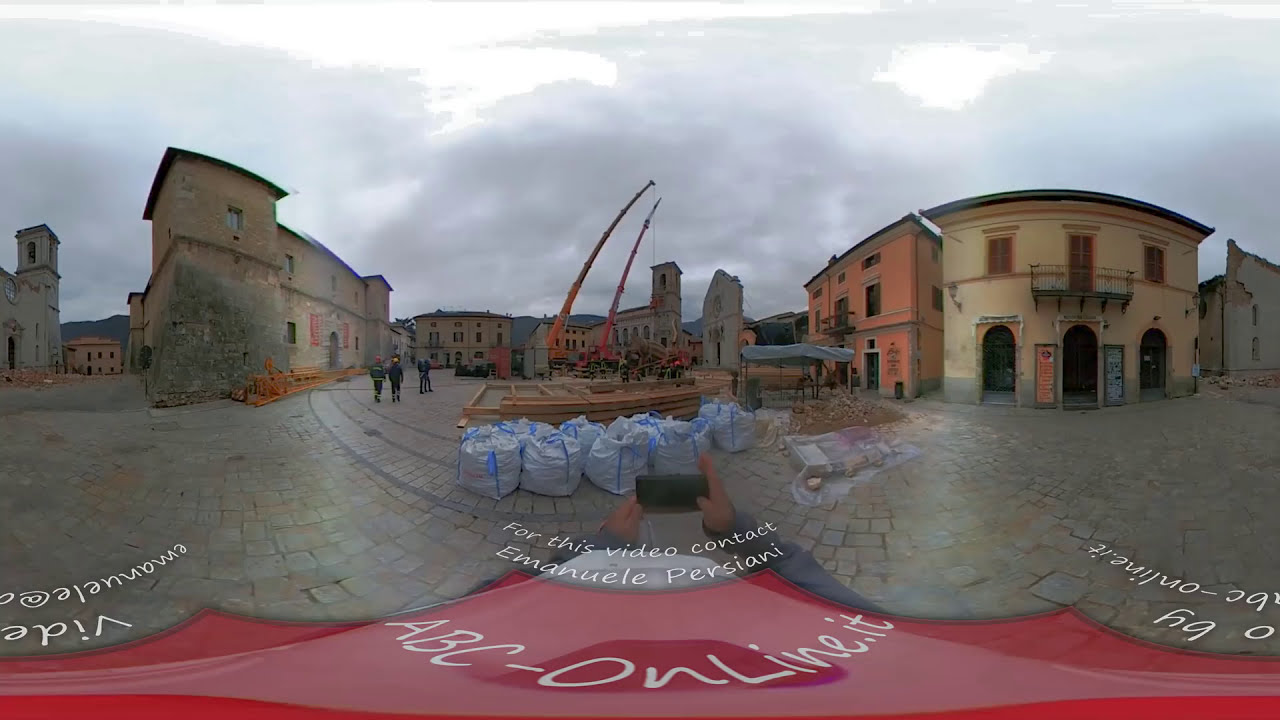This is a panoramic color photograph with a fisheye lens effect, giving it a slightly distorted appearance. The image is composed of three sections blended together seamlessly. On the left, there's a two-story villa adorned in beige with a stone courtyard evocative of a charming Tuscany setting. Notably, one of these buildings features a tower with an arched window at the top. Central to the photograph is an active construction site, evident by dark-clad workers in yellow helmets, large gray-blue trash bags, and wooden framing scattered around. Orange cranes loom in the background, highlighting ongoing development in this large plaza. Especially noticeable are the text details: "For this video, contact Emanuel Persiani" and "abc-online.it" in white, thin lettering on a red strip at the bottom of the image. To the right, a pair of two-story villas appear, one in yellow stucco with a walkout balcony and a rounded wall, the other in a similar orange shade, both set against a backdrop of green tile pavers. The scene is enveloped by structures reminiscent of a quaint European village, with cobblestone streets and an overcast sky completing the tableau.